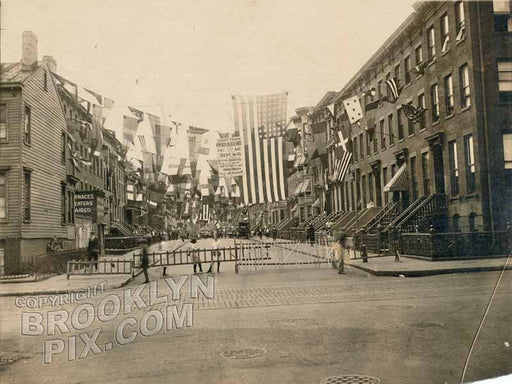This vintage black-and-white photograph, slightly sepia-toned, captures a bustling urban scene from olden-day America. It features brick and wooden terrace houses on both sides of a prominent boulevard, running from the foreground into the distance. The left and right sides of the image are framed by these buildings, which possess awnings and metal railings leading up to elevated entrances. The street is adorned with a variety of flags from different nations, arching overhead between the buildings. A prominent, giant American flag with stars in the upper right-hand corner and stripes dominates the center of the flag display. In the foreground, several men and women are carrying a wooden ladder across the road, while smaller figures and possibly a vehicle can be seen in the distant background, suggesting a lively street party. The image, marked with a "copyright brooklynpix.com" watermark in the bottom left corner, immortalizes a dynamic and richly detailed snapshot of a bygone era.